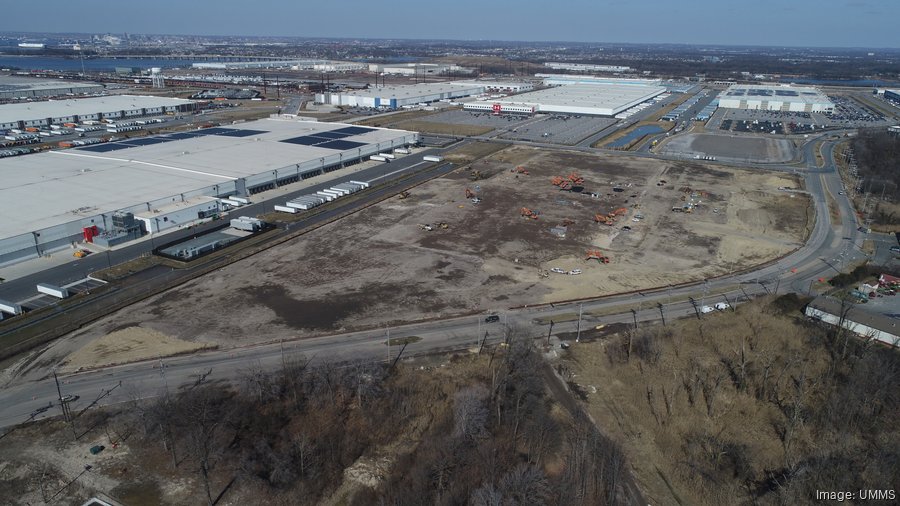This high-resolution aerial drone photograph, taken from an elevation of approximately 100 to 200 feet, showcases a sprawling industrial complex populated with several vast warehouses. Dominating the foreground, a wide road bisects the scene, curving from the left to run parallel to the bottom edge before veering towards a large, prominent white-roofed warehouse. This principal building is not tall but spreads expansively, its roof adorned with neatly arranged solar panels. Surrounding this warehouse, numerous white semi-truck trailers are uniformly parked, with several trailers positioned at loading docks in the rear. Adjacent to these facilities is a vacant lot, appearing to be under construction, populated with various pieces of construction equipment.

Beyond this main warehouse, the image reveals additional large white-roofed warehouses, each with distinctive roof features of blue, red, and beige hues. These secondary structures are bordered by extensive parking lots crammed with hundreds of vehicles, indicating spaces designated for employee parking. On the rightmost side, another warehouse starkly stands out with its vast, white expanse and lack of truck activity, suggesting it might serve a manufacturing purpose.

In the distant background, the picture captures a faint silhouette of a city skyline beyond a body of water, possibly a river, traversed by an elongated bridge. The image is bathed in clear sunlight under a bright blue sky, embodying a detailed and expansive view of this bustling industrial zone. The bottom right corner of the image is marked with the text, "Image, U-M-M-S," providing a subtle watermark to this detailed photographic capture.